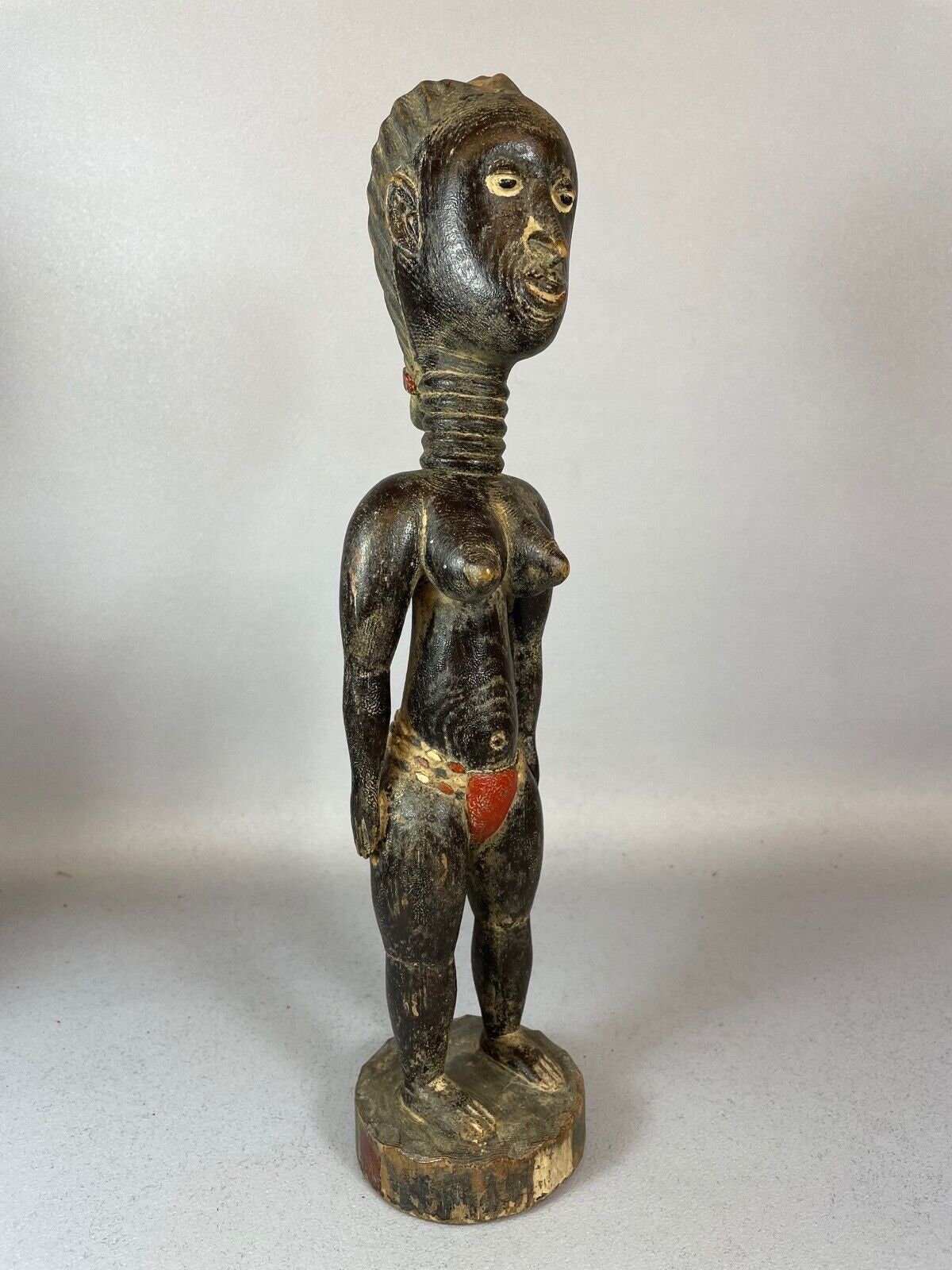The image displays a detailed wooden statue, appearing to be an ancient artifact from an African tribe. The statue is expertly carved from a dark wood and portrays a woman with a rounded head and hair that stands straight out. Her neck is elongated and adorned with multiple rings resembling chokers, possibly signifying an extended neck. The woman is topless, exposing her breasts, and her torso is covered with intricate tattoos. She is dressed in a loincloth, fastened by a belt that is designed to appear bejeweled. The statue stands barefoot on a circular base, ensuring its stability. The image captures the sculpture in a clear and bright setting, against a plain white background, much like a photograph taken to highlight a museum piece. No additional objects or text are present in the image, allowing viewers to fully appreciate the craftsmanship and cultural detail of the statue.